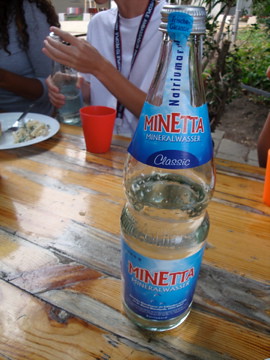A highly detailed photograph captures a bottle of Mineta mineral water resting on a polished, multi-toned wooden table. The table, featuring various shades of gray and brown with visible knots and a glossy lacquer, is set outdoors amidst a background of lush green plants and bushes. The clear, tall bottle of water, half full, features distinctive blue labels with red text that reads “Mineta” on both the top and bottom halves. Underneath "Mineta," the label is inscribed with "Mineral Wasser. Classic!" in white text. The bottle is capped with a sleek silver twist cap. In the background, on the upper left corner of the image, there is a plate of food, a red cup, and another bottle of water held by an individual wearing a white shirt and a lanyard, though their face is not visible. A second person is seated next to them at the same outdoor table.